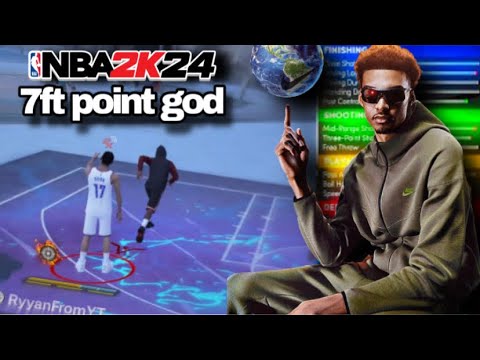The image appears to be a screenshot, possibly taken from a computer or TV screen, as indicated by the black borders at the top and bottom framing a rectangular picture. At the center of the image, there is a horizontal display featuring two sections.

On the left side, there is a portrayal of video game basketball players, with one player in a white and blue uniform and another in black. Above this, text reads: "NBA 2K24, 7 foot point guard."

On the right side, there is an image of a black man seated in a chair, facing diagonally towards the left. He is wearing an olive green tracksuit adorned with a Nike symbol on the chest. The man has reddish-tinted hair and is wearing sunglasses. He holds his right hand up, balancing a globe of the Earth on one finger, in a poised manner. His facial expression is neutral, and he gazes directly at the camera. The background behind him is illuminated with a colorful array of lights in green, blue, yellow, and red.